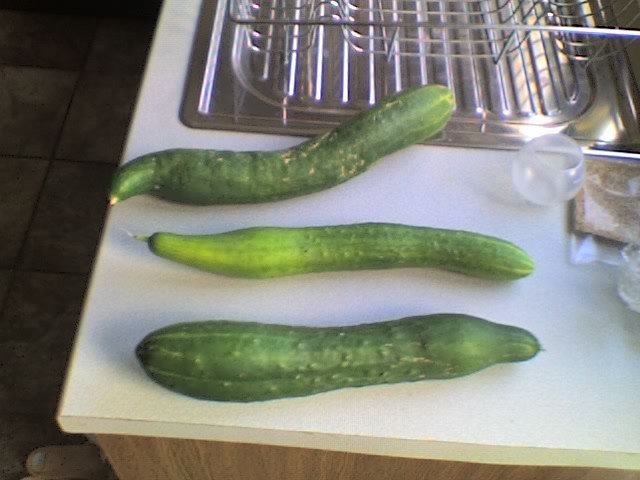The photograph captures a well-lit kitchen scene with a detailed view of the countertop and surrounding elements. On the off-white, vinyl countertop in the foreground, there are three misshapen, green cucumbers (initially mistaken for zucchini), each exhibiting unique and irregular shapes. The largest cucumber at the bottom varies in girth, with a medium green hue, the second is long and thin with a gradient from lime green to medium green, and the third, most peculiar, has an S-shaped curve with noticeable markings that could indicate growth-related damage. 

Above the cucumbers is a metallic, stainless steel dish rack situated over a chrome-colored sink that strays out of the frame. To the right of the sink, a glass and a package, possibly containing grain, sit on the counter. On the far left edge of the photograph, part of a tile floor with large off-white tiles and dark grout is visible. The scene conveys an everyday kitchen setup, ready for meal preparation, with ingredients and utensils neatly arranged.